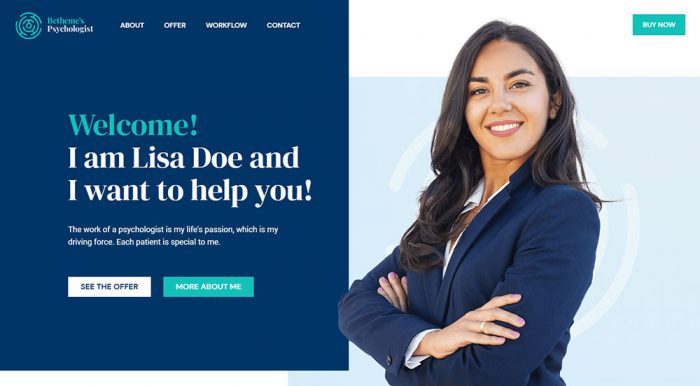The image features a visually striking blue background on the left side, accentuated by a white section on the left that includes a blue circle and text at the top-left corner. Prominently displayed in white font to the right of the blue background are the menu options: About, Offer, Workflow, and Contact. Below this, in blue font, the text reads "Welcome," followed by a white font introduction: "I am Lisa Doe and I want to help you." Additionally, there is smaller text that elaborates: "The work of a psychologist is my life's passion, which is my driving force. Each patient is special to me."

A white square with blue text invites viewers to "See the Offer," and a green square with white text prompts them to "More About Me." Centrally, the image showcases a white female with brown hair, wearing a white collared shirt and a blue jacket. She also has a ring on her left finger. The background behind her is predominantly blue, featuring a subtle greyish-line circle for added texture.

In the top right corner, another green square with blue lettering reads "Buy Now." The overall layout sits on a white background that continues both above and below the central picture, creating a clean and professional appearance.